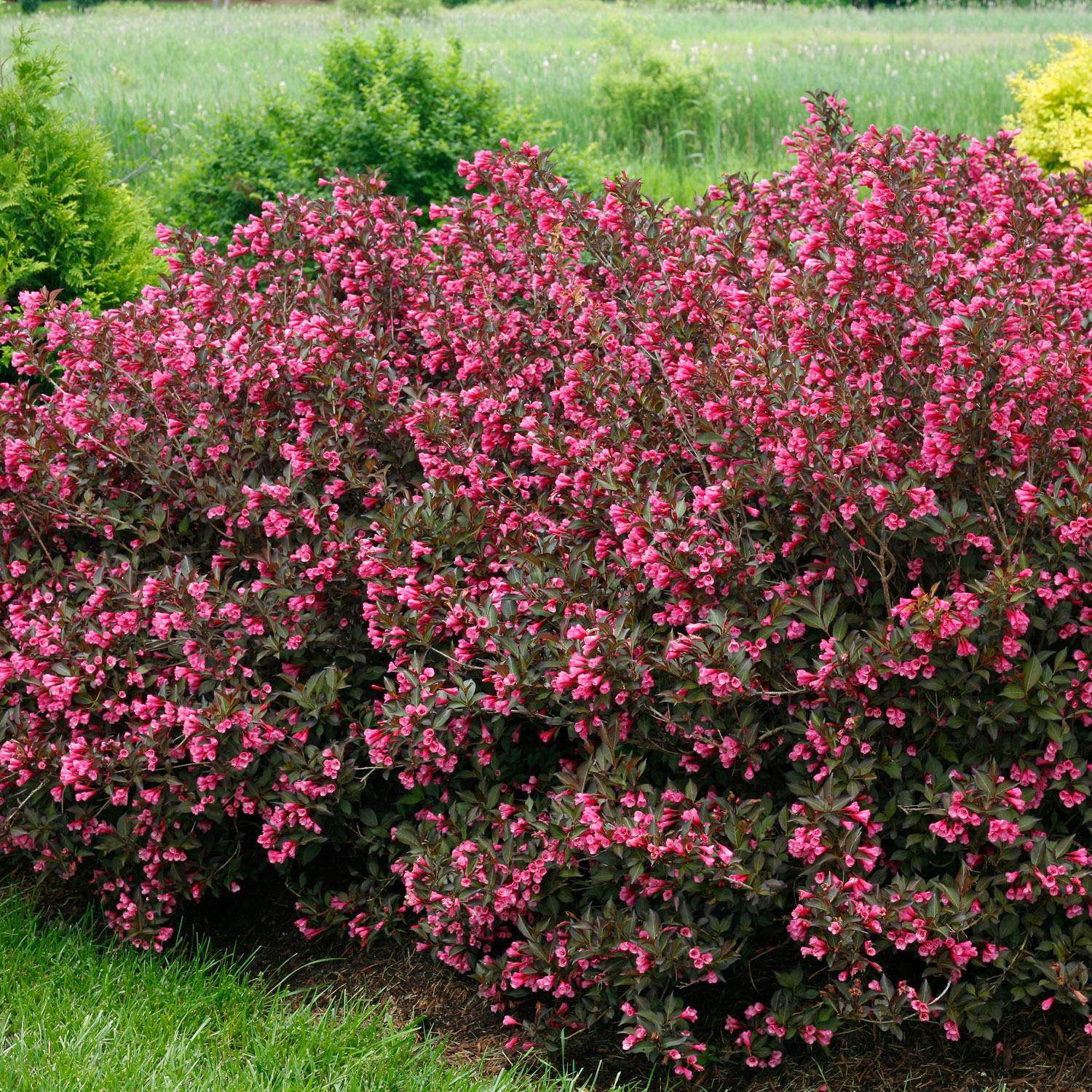The image showcases a vibrant nature scene with a large, densely-packed bush adorned with bright pink flowers as the main focal point. The pink flowers cover the bush from the left-hand side, spanning almost the entire width of the image, with the most abundant cluster at the top and increasingly visible dark green leaves towards the bottom. In the lower left-hand corner, a small patch of green grass is noticeable, and towards the bottom, patches of dirt are visible beneath the bush and in the bottom right corner. In the background, a field of green grass is dotted with small, purely green bushes, and on the upper right side, a bright yellow plant stands out. The overall scene is lively and colorful, with the mesmerizing pink-flowered bush stretching across the image and creating a striking contrast against the greens and yellows of the surrounding foliage.